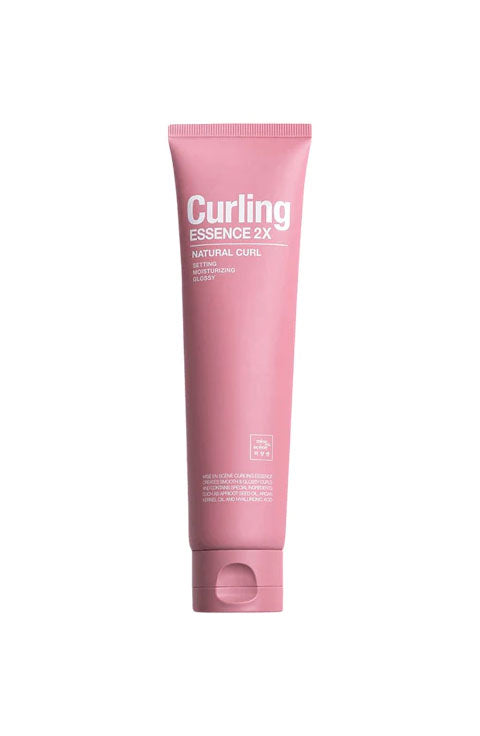This image showcases a simplistic, product shot of a pink squeeze tube standing upright on a white background, designed as a styling product or lotion. The tube, which resembles a setting moisturizer or glossy product, features white sans serif lettering. Prominently displayed at the top are the large words "Curling Essence 2X" followed by "Natural Curl." Additional, smaller text below these headings and at the bottom of the tube details further product information, likely ingredients or claims of effectiveness, though this text is too small to read clearly. The tube, a dusty pink color, has a flip-top cap at its base, facilitating easy access, especially useful if hands are wet. This minimal packaging style emphasizes functionality and practicality for styling purposes.